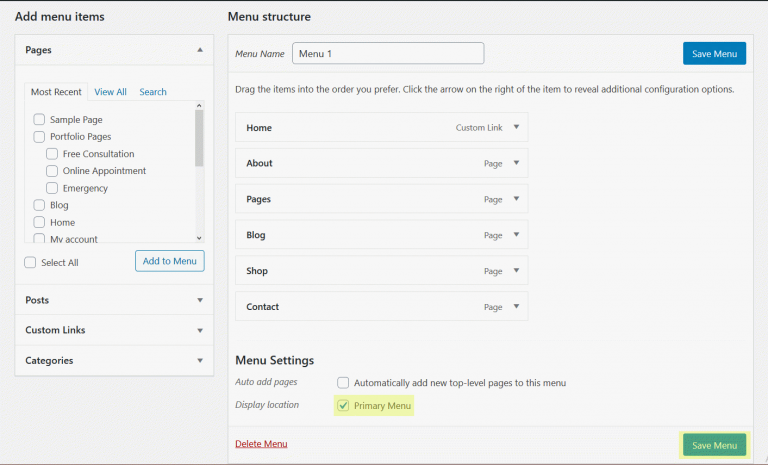### Caption:
A detailed view of a menu management interface within a web app or program. On the left side, there is a column labeled "Add Menu Items" featuring sections like "Pages," "Posts," "Custom Links," and "Categories," each with various options for item selection such as "Sample Pages," "Portfolio Pages," "Free Consultation," "Online Appointment," "Emergency," "Blog," "Home," and "My Account." None of these options are currently selected. 

Below the "Pages" section, there's an option to "Select All" and a button to "Add to Menu," both of which remain unchecked. More options with dropdown menus like "Posts," "Custom Links," and "Categories" are present but not expanded. 

Moving to the center, the "Menu Structure" section is featured prominently. It includes a text field labeled "Menu Name," which is currently set to "Menu 1," suggesting this is the title of the menu. A blue button labeled "Save Menu" is present underneath. Instructions below this field prompt users to "Drag the items into the order you prefer" and to "Click the arrow on the right of an item to reveal additional configuration options."

The menu items listed under "Menu Structure" are: "Home" (a custom link with a dropdown menu), "About" (a page with a dropdown menu), followed by "Pages," "Blog," "Shop," and "Contact," each with a page designation and an associated dropdown menu.

At the bottom, there's a "Menu Settings" section. The option "Auto Add Pages" is available but unchecked, offering to automatically add new top-level pages to the menu. The "Display Location" is checked and highlighted in a yellowish-green color, indicating this menu is set as the "Primary Menu." Finally, options to "Delete Menu" and "Save Menu" are displayed in red text at the bottom.